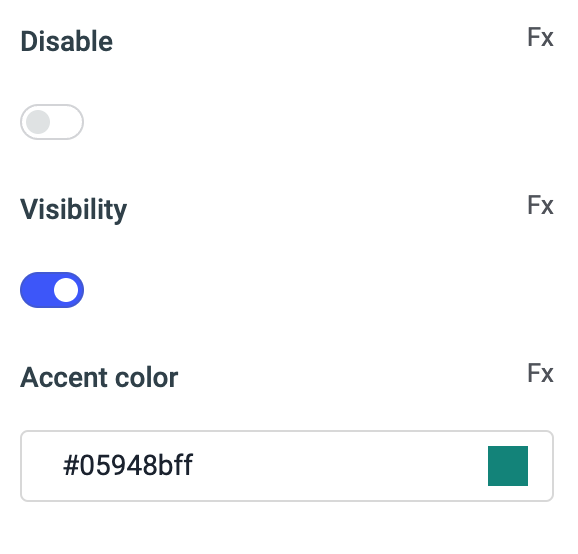This image features a user interface design with a white background and black text. At the top left corner, the text reads "Disable." Below this text is a toggle switch that is currently turned off, indicated by its gray color and leftward position.

Directly to the right of the "Disable" section, the text "FX" is displayed. The second option underneath is labeled "Visibility," also on the left side. Adjacent to this label is another toggle switch. This switch is turned on, signified by its blue color and rightward position.

At the bottom of the image, the text "Accent Color" is written, with the corresponding label "FX" on the right side. Below "Accent Color" is a rectangular box displaying a slightly dark green color. Within this box, the hexadecimal color code "#05948BFF" is written.